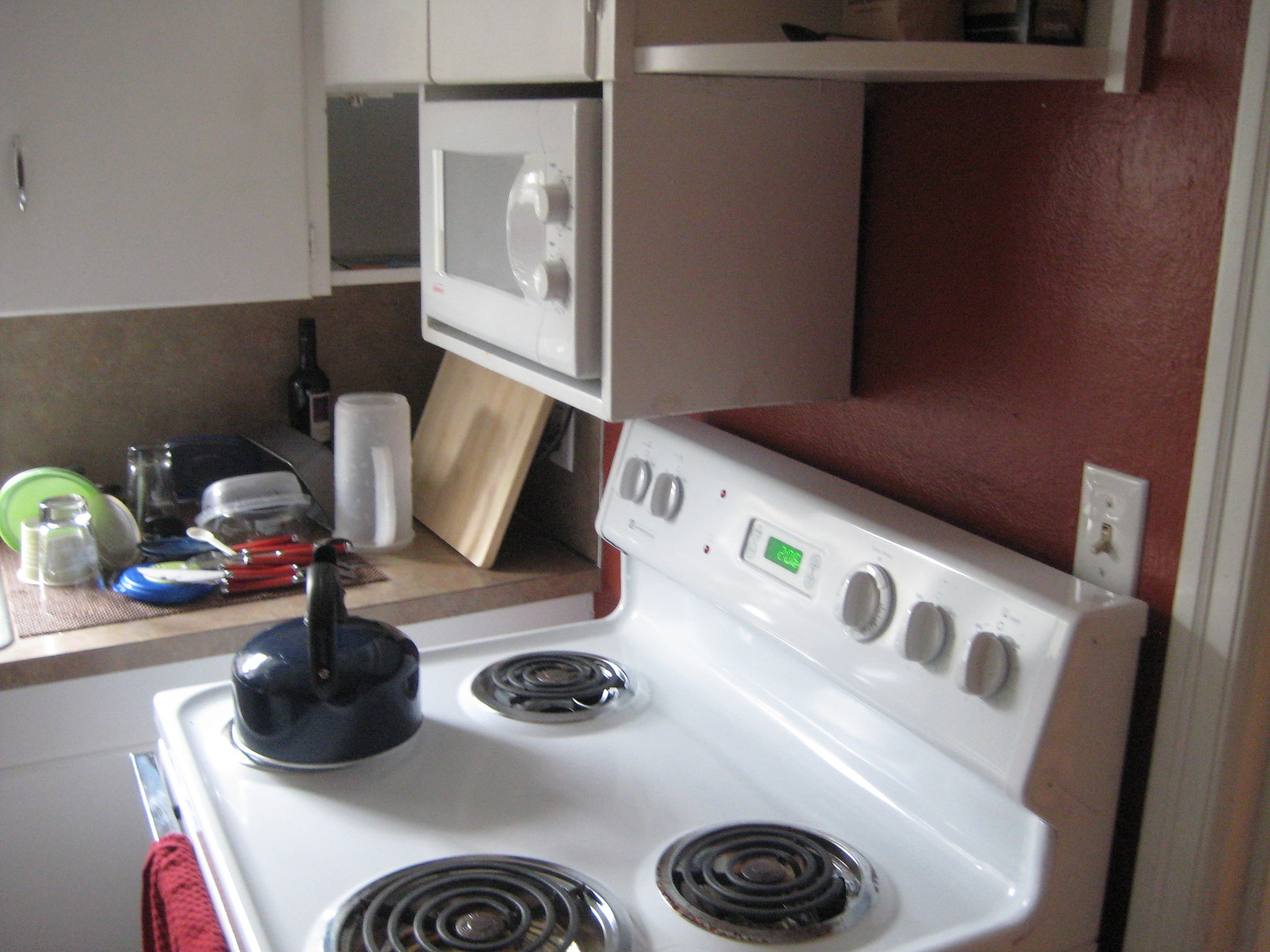The image showcases a kitchen corner featuring a stove as the central element. Situated on the bottom left burner, there is a distinctive blue kettle. Above the stove, a pristine white microwave is mounted, seamlessly blending with the white cabinetry that adorns the upper and lower sections of the kitchen. The walls provide a striking contrast, painted in a bold red hue, adding vibrancy to the predominantly white decor. A light switch is also visible on the red wall, contributing to the functional aspects of the space.